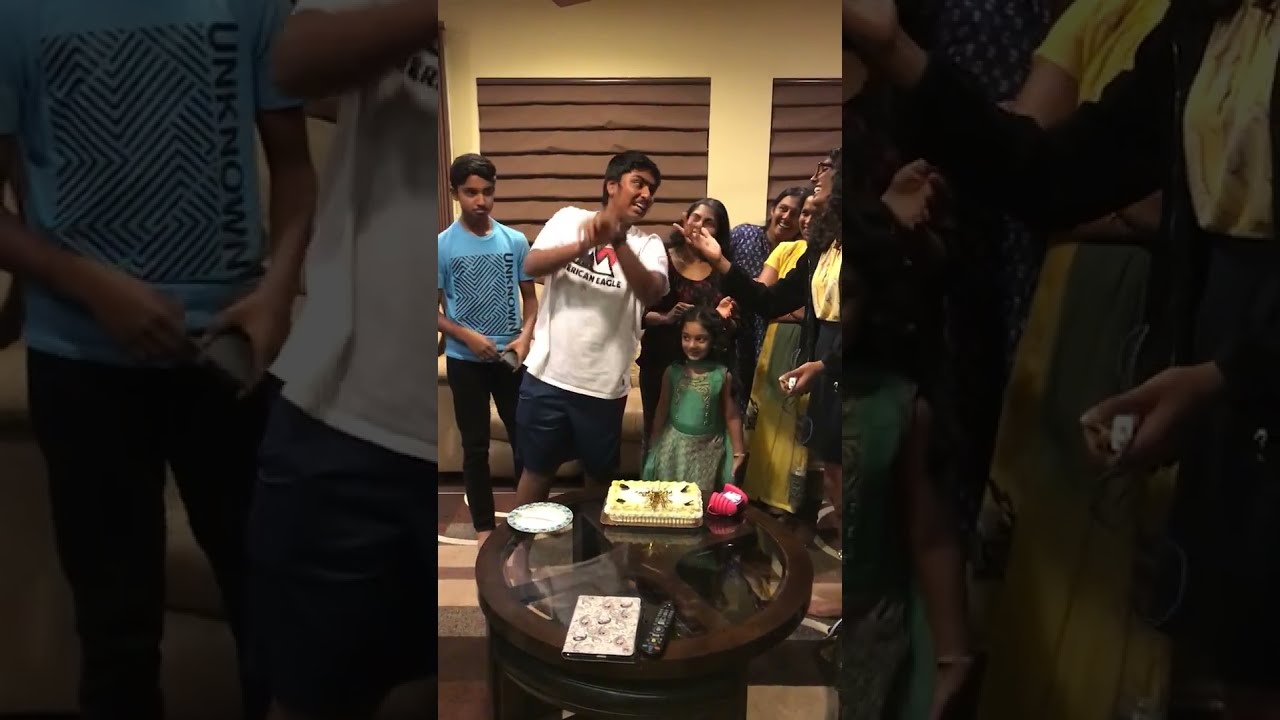This photograph captures a lively moment featuring a group of Indian descent in a cozy living room. Central to the image is a circular wooden table with a glass top, cluttered with various items including a remote control, a decorative ring binder, a small electronic device in a case, a pink purse, and a paper plate with a cake on it. The table's placement and its contents suggest it is a focal point in the room.

Behind the table stands a diverse group of individuals, including two boys, five women, and a young girl, all of whom seem to be enthralled by something. The boy on the left is about 17 or 18 years old, wearing a white T-shirt, possibly from American Eagle, and blue shorts. He holds something up to his mouth, perhaps taking a bite, while his hands obscure his face. Next to him is a younger boy dressed in a turquoise short-sleeved t-shirt and long black pants.

Flanking the boys are four women, each dressed in distinctive outfits. From left to right: one woman in a dark top with red and black hues, another in a striking navy blue dress, another in a vibrant yellow sari, and on the far right, a woman mostly cropped out of the shot, distinguished by her black cardigan. In front of this line of people stands a little girl, around six years old, in a kelly-green dress. Everyone appears amused, their attention possibly diverted by the boy in the white T-shirt.

Adding a personalized touch to the environment, the backdrop reveals a brown and yellow wall, hinting at a warm and inviting household. The scene suggests a close-knit family gathering, with members interacting expressively and joyfully.